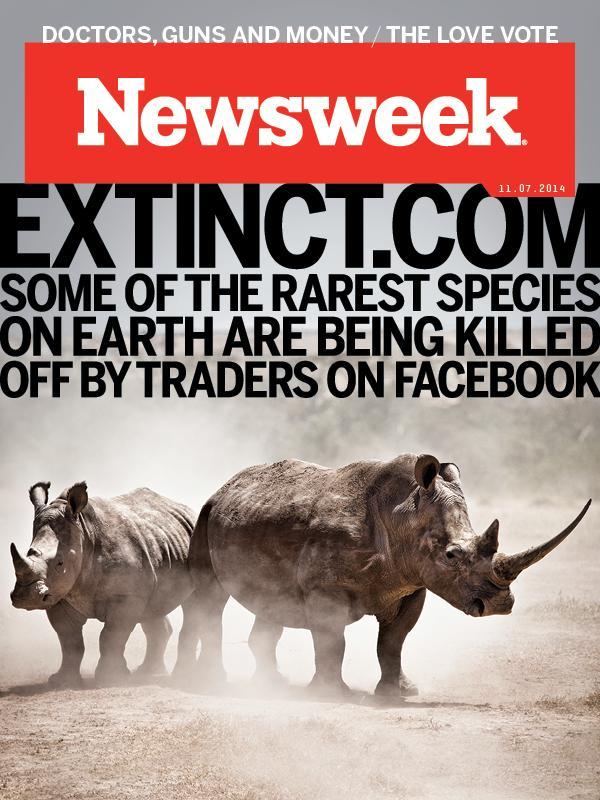This is a detailed description of the Newsweek cover for November 7, 2014. The background is predominantly grey, accentuating the cover's headline: "DOCTORS, GUNS, AND MONEY, THE LOVE VOTE," which is written in bold white letters. Below this headline, a red banner showcases the Newsweek logo in white, using a distinct font. The issue's publication date, "11.07.2014," appears in white lettering just beneath the logo. Following this, in bold black uppercase letters, the text "EXTINCT.COM" is prominently displayed. Just below, a smaller caption reads, "Some of the rarest species on Earth are being killed off by traders on Facebook," also in bold black capital letters. The lower section of the cover features an image of two rhinoceroses standing on sandy terrain under a moody, grey sky. The rhinoceroses are positioned with their sides leaning into one another; one has a small horn paired with a notably long horn, while the other has just one small horn, highlighting their distinct physical characteristics.